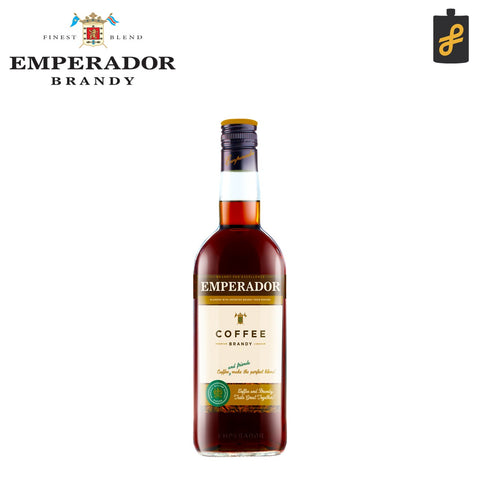This image is an advertisement showcasing a bottle of Emperador Coffee Brandy on a white backdrop. In the upper left-hand corner, the logo features a family crest with two flags and the text "Finest Blend" above "Emperador" in black capital letters. To the right-hand corner, a black flask with a golden-style ampersand is visible. The centerpiece is a coffee-brown colored bottle of brandy with a dark purple screw cap and white highlights on its sides. The label reads "Emperador" at the top, followed by a gold horizontal line, and below it, a creamy white background labeled "Coffee Brandy." Additional text is present below but is not legible. The overall presentation emphasizes the luxurious and crafted nature of the liqueur.